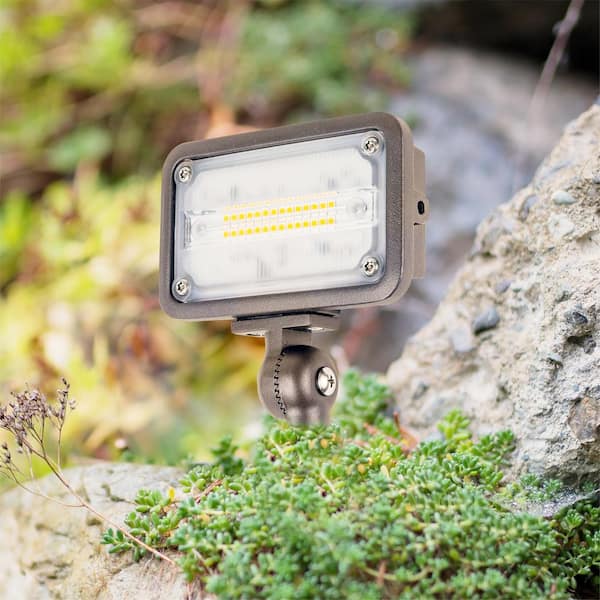The image showcases a close-up shot of a rectangular electronic device that resembles a trail camera or an LED light on a swivel stand. The device is encased in brushed steel or silver-colored casing with a screen secured by four screws, one in each corner. It has yellow writing on the screen. This device is prominently placed between two chalky, white-colored rocks covered with green moss and scattered yellow and green foliage, suggesting an outdoor, wooded setting. The detailed texture of the rough, honed rocks is visible, with various pebbles protruding from them. Some cobwebs are also noted in the bottom right corner and extending onto one of the rocks. The background is blurred, emphasizing the natural environment and hinting at foliage and possibly a wooded area beyond the rocks.